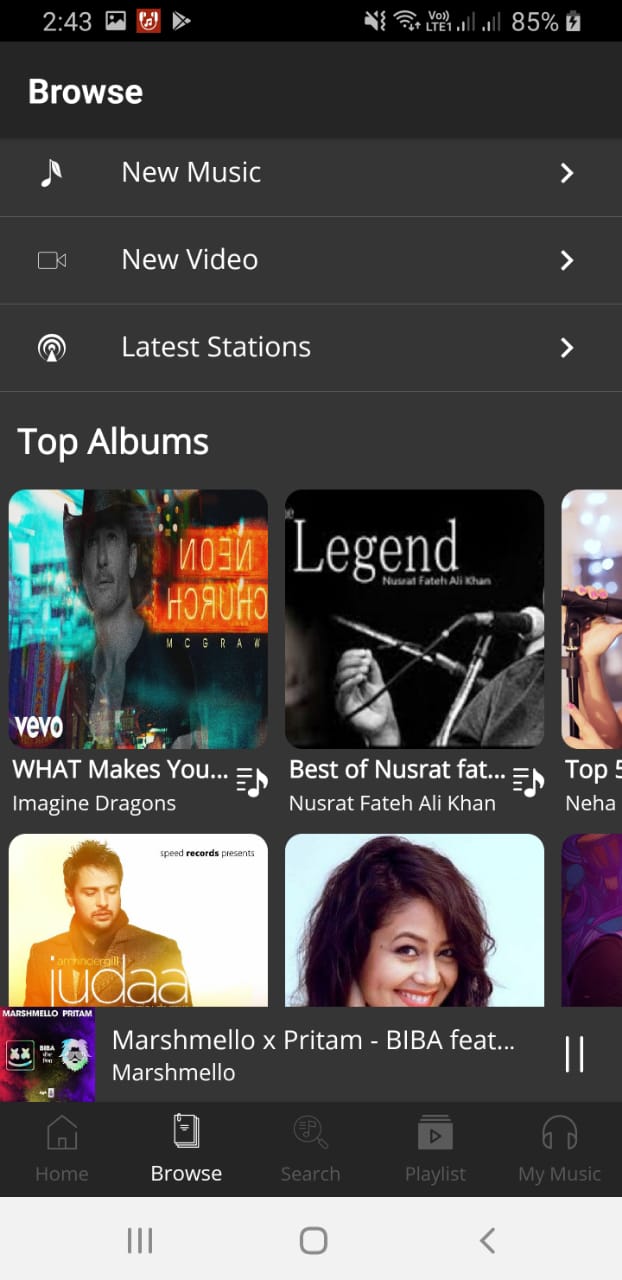The image showcases a detailed screenshot of a music app displayed on a mobile phone. At the top, there is a black border featuring the text "243" alongside an images icon, a red headphones icon, and a Google Play icon. In the upper right corner, various icons are visible: a no sound icon, a Wi-Fi icon with up and down arrows, the text "VOLTE 1" next to two data icons, and a battery icon indicating 85% charge with a charging symbol.

Below this black border, in a gray section, the word "Browse" is displayed in white text. This section includes several navigation options depicted with icons and labels: a musical note icon labeled "New Music" with a right-facing arrow, a video camera icon labeled "New Video" with a right-facing arrow, and a target-like icon labeled "Lightest Stations" with a right-facing arrow.

Further down are listings of top albums highlighted with album cover images and titles. Specific albums mentioned are "What Makes You" by Imagine Dragons, "The Best of Nusrat Fateh Ali Khan" by Nusrat Fateh Ali Khan, and an unspecified album featuring an image of a woman with brown hair and an image of a man in a brown jacket labeled "Judah." There is also mention of "Marshmello x Pritam BIBA feat Marshmello."

At the bottom of the screen, a navigation bar indicates different selectable options: Home, Browse, Search, Playlist, and My Music, with "Browse" currently selected.